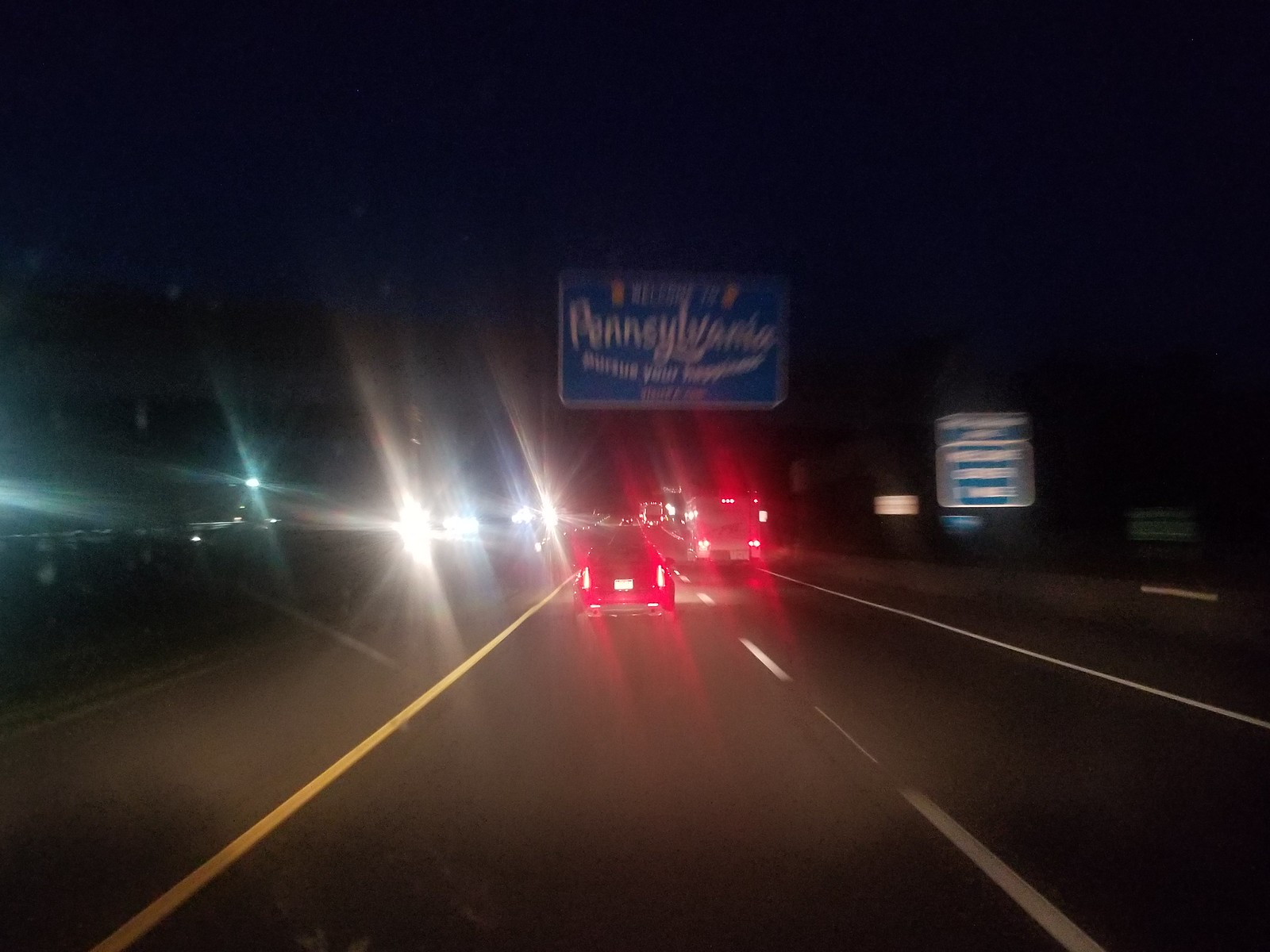A nighttime photograph depicts a multi-lane highway observed from a vehicle's windshield. The image appears blurry, with notable features of the highway including a yellow line on the leftmost side, a dotted white line in the middle, and a solid white line on the right. Two vehicles are directly ahead, their red taillights emitting a noticeable glare that streaks vertically, obscuring the vehicles themselves. On the left side of the photograph, three bright white lights add to the overall glare and distortion. A blue sign with white lettering is visible at the top of the image, reading "Welcome to Pennsylvania," though the text beneath is illegible due to the blur. An additional blurred sign is present on the right-hand side of the highway, its contents also unreadable. The overall composition conveys the challenges of nighttime driving under conditions that impair visibility.